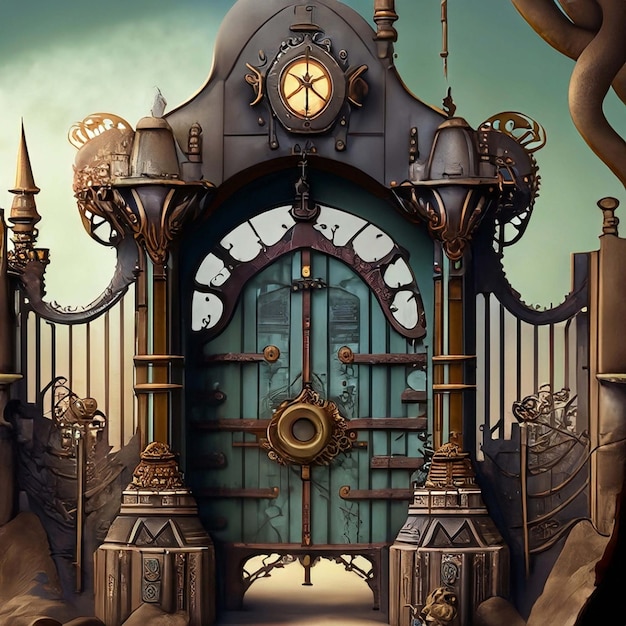This detailed computer-generated drawing features an elaborate outdoor gate set against a grayish sky with white clouds. The gate itself has a distinct steampunk feel, characterized by intricate, non-functional gadgets and an overall metallic design. The central architectural element is an iron gate with an arched top, flanked by two decorative metal pillars. The pillars have bases, tapering bodies, and ornate tops adorned with tiny points.

The gate comprises light blue metal, and the arched section features a light source. Below the arch, there's a pair of green doors, accentuated with a large, circular bronze door knocker. Situated above the doors are small openings, possibly windows. Wrought iron elements extend on either side, resembling a curved fence adorned with vertical bars.

The upper left corner of the image showcases a star spire element, while the upper right corner reveals several bronze-colored pipes. This sophisticated gate design includes detailed horizontal and vertical metal sections and mirrors a fence structure with vertical projections. Overall, this steampunk-inspired scene captures the intricate blend of ornamental and mechanical design elements.